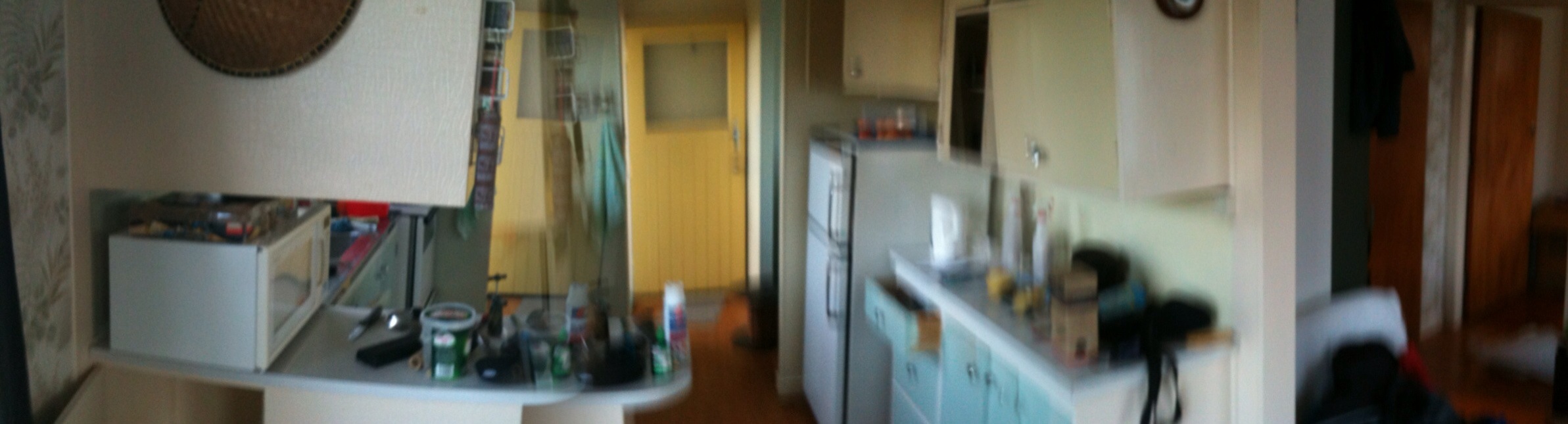The photograph is an expansive, panoramic shot of a kitchen taken with a smartphone, resulting in a slightly curved, horizontal stretch across the image. The kitchen features light blue lower cabinets and beige upper cabinets, with countertops that are covered in a multitude of items, creating a cluttered appearance. A white microwave sits prominently on the left side of the counter. The countertops and items are slightly out of focus, contributing to a somewhat blurry image quality.

In this wide-angle view, a white refrigerator with large handles is visible towards the right, positioned behind a side bar area. The image extends into another room on the far right, though the details are indistinct due to low resolution; visible elements include a white marble-like pillar, a dark brown mahogany door, and a piece of white furniture that could be part of a bed or a chair. The photograph also shows some glitching, particularly around a yellow door with a glass square cutout that appears split and out of focus, indicating a quick panorama shot. The floor appears to be hardwood, and there's mention of a white countertop amidst the clutter.